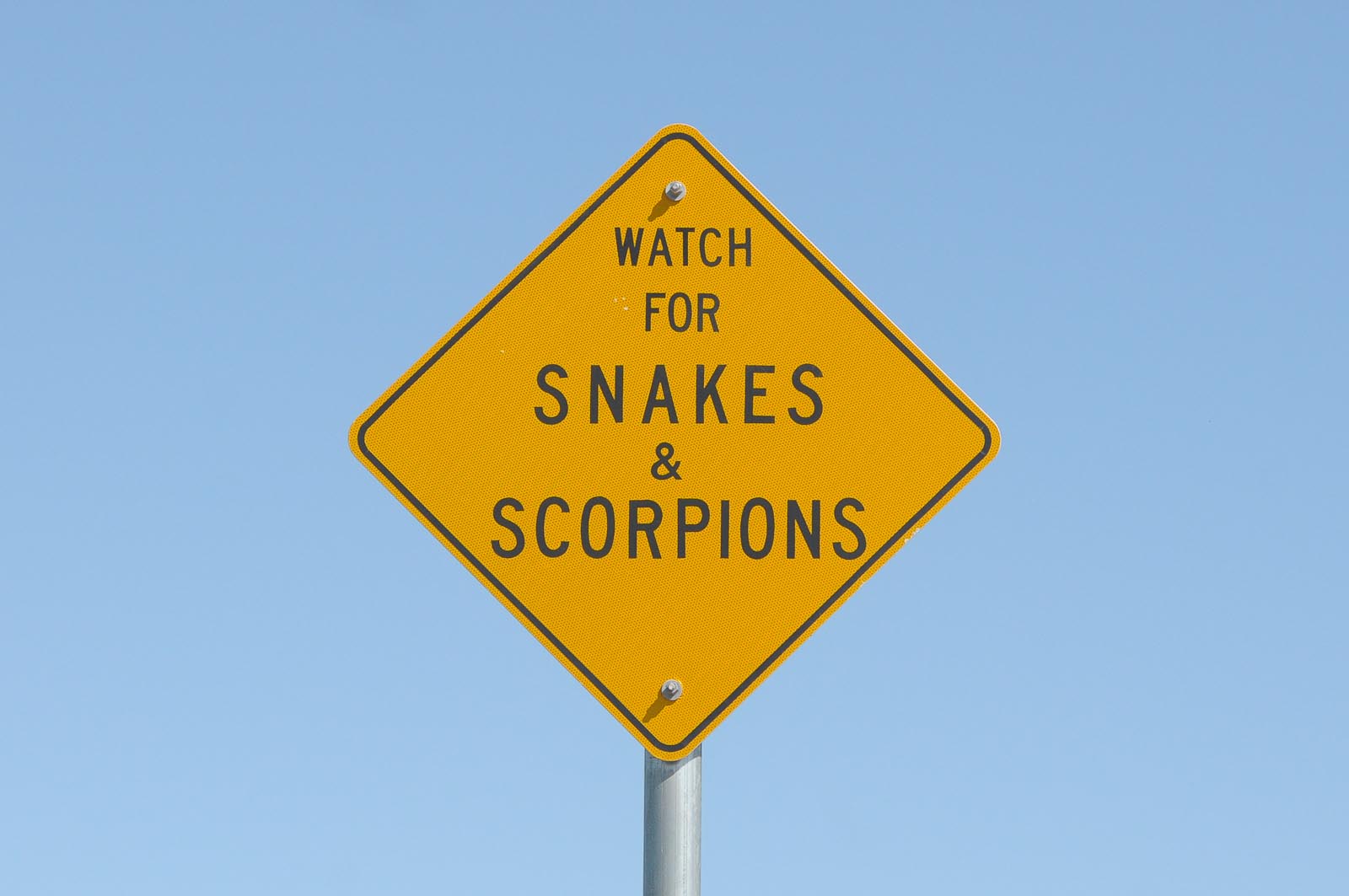In the image, there is an alert sign set against a vibrant blue background, which could either depict a clear blue sky or a digital backdrop. The sign itself is diamond-shaped and yellow, outlined with a bold black border. Centered on the sign, the warning message "WATCH FOR SNAKES AND SCORPIONS" is prominently displayed in dark lettering, either in black or a very dark brown. The conjunction "AND" is symbolized by an ampersand (&) instead of the full word. The sign is affixed to a sturdy silver pole with two silver screws, each secured with washers, ensuring the sign remains firmly in place. This detailed warning sign is crucial for informing and protecting individuals in the area.